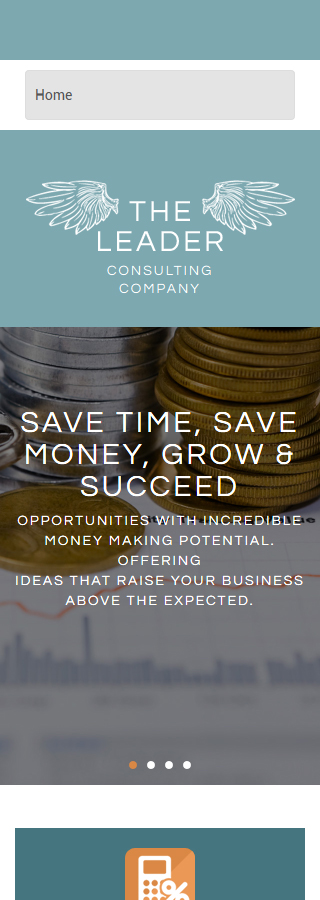This image is a screenshot featuring branding elements from the Southworth Consulting Company. The top section of the image is dominated by a horizontal aqua-colored bar extending from the left to the right edge. Directly below this is a grayish bar that also spans the width of the image, with center-justified text. The word "Home" is displayed in gray font on the left-hand side of this bar.

Beneath these bars, the main content area is highlighted. Here, another horizontal bar, matching the aqua color of the top bar, features prominently. This bar contains the text "The Leader Consulting Company," where the words "The Leader" are in a larger font, with "The" positioned directly above "Leader." Stylized wings are intricately integrated next to the letters "T" and "E" in "The." Positioned below this aqua bar is an image depicting a stack of coins, reinforcing a sense of financial expertise or economic success associated with the consulting company.